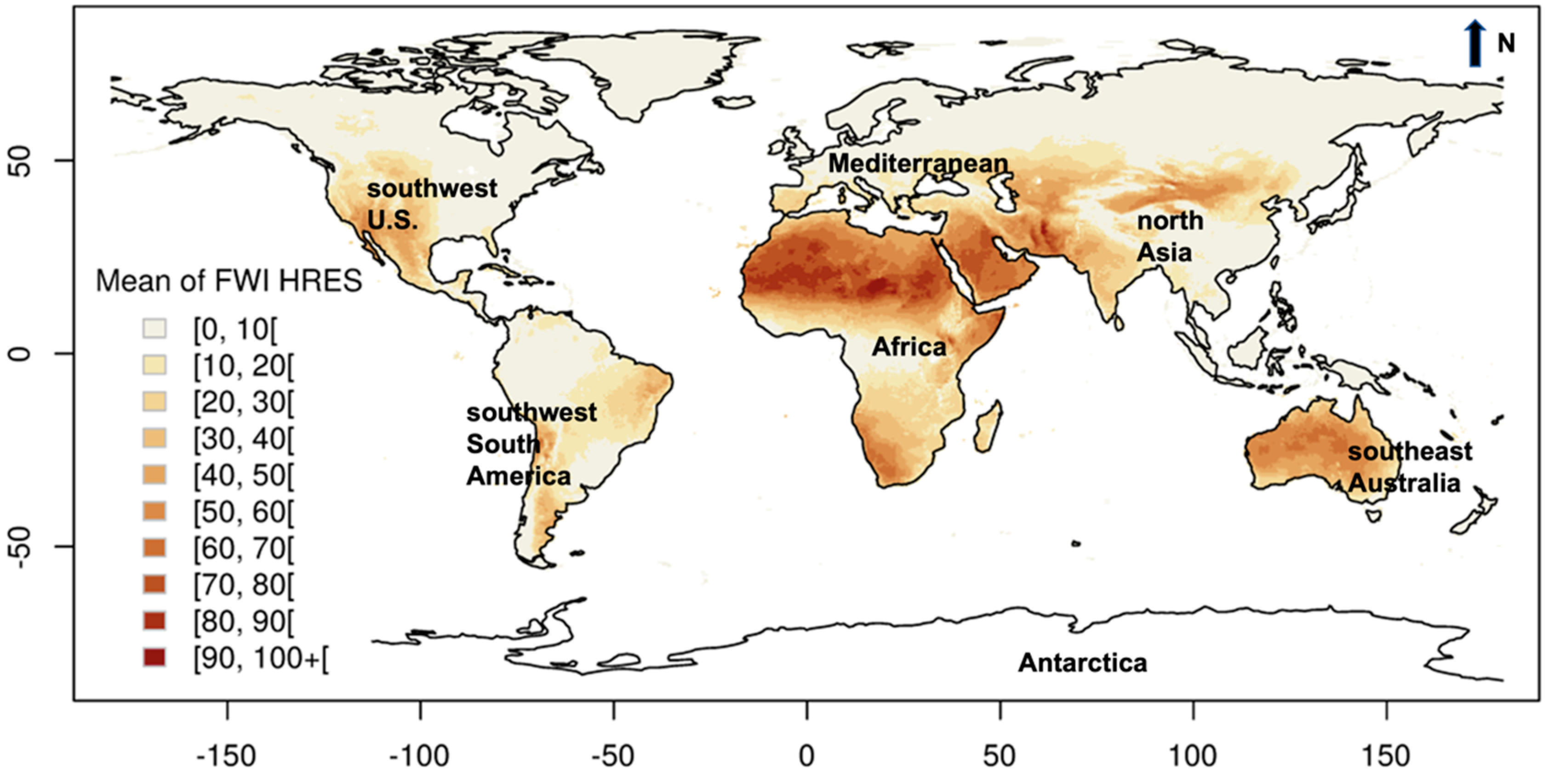This image depicts a rectangular world map prominently featuring detailed geographical and navigational information. On the left side, a vertical scale marks the latitude with demarcations at -50 degrees, 0 degrees, and 50 degrees. Along the bottom edge, a horizontal scale displays the longitude with marked intervals at -150 degrees, -100 degrees, -50 degrees, 0 degrees, 50 degrees, 100 degrees, and 150 degrees. Positioned in the top right corner is a black arrow pointing upwards, accompanied by the letter 'N', indicating the direction of north.

A color-coded key is also present on the map, which explains the varying hues used to represent the land masses. The land masses are shaded in a gradient ranging from white to medium brown. This gradient is labeled under the scale titled "Mean of FWIHRES," and the key provides a detailed explanation of what each shade signifies.